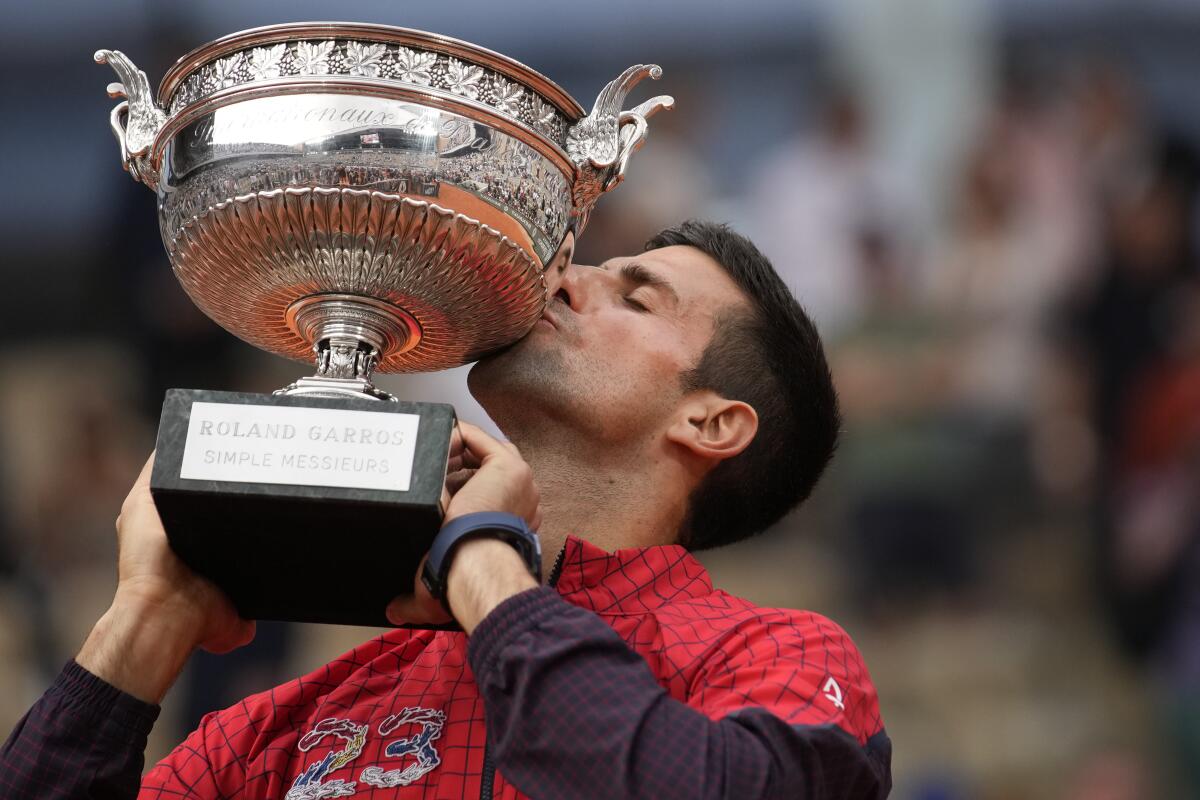In this photograph, a man, believed to be tennis player Novak Djokovic, is captured holding and kissing a prestigious trophy at face level with both hands. The trophy features a wide, ornate silver bowl with intricate designs and wing-like shapes flaring from its sides. The base of the trophy is adorned with a metallic plaque that reads "Roland Garros" and "Simple Messieurs," indicative of a major tennis tournament held on clay courts in Paris. The man is dressed in a striking red and black checkered jersey, bearing the number 23 in red, yellow, blue, and white on the right side of his chest—likely signifying the number of major tournaments he has won. His short brown hair is visible as he tilts his head slightly upwards, eyes closed in a moment of triumph. A reflective crowd can be seen on the surface of the silver cup, while the background of the image remains blurred, drawing focus to the emotional celebration. Additionally, he is wearing a wristband and a watch, emphasizing his distinctive style.